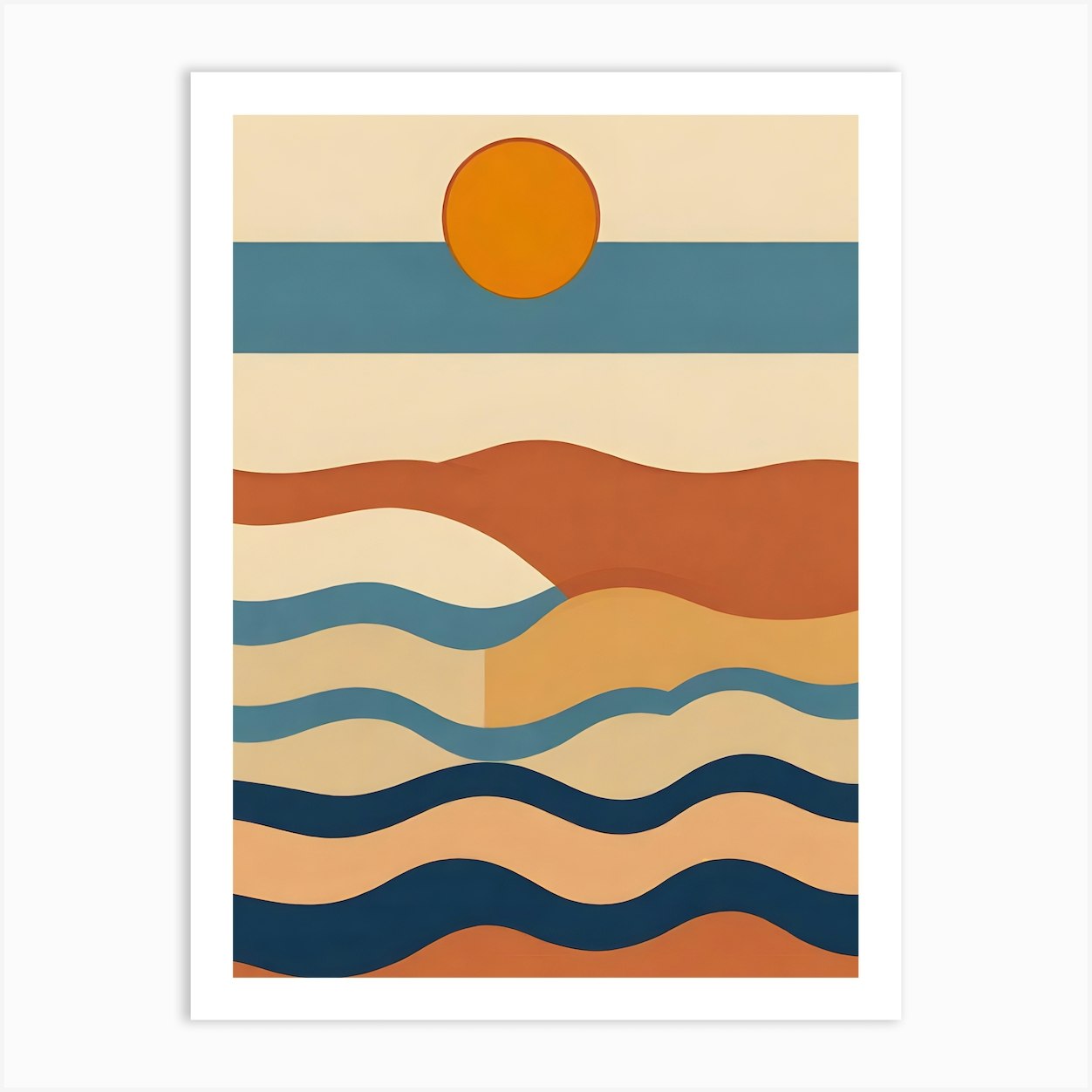This piece is a modern art interpretation of a beach scene, blending abstract and vintage elements into a unique design. Dominated by layers of various colors, the artwork features a sequence of thick, undulating waves covering the lower half of the image. These waves are rendered in multiple hues, including dark turquoise, rusty orange, beige, brown, and different shades of blue, capturing the essence of reflected sunlight and water. Above the waves, a simple depiction of the sky is represented by a blue horizontal line, crowned by a striking orange sun. The sun, a dark rusty orange circle, sits prominently atop the blue line, encapsulating the moment of either sunset or sunrise. The entire background is a minimalist beige, framed by a white border, enhancing the modern and abstract feel of the piece. The juxtaposition of color layers suggests a serene beach at sunset viewed through an abstract, layered lens.